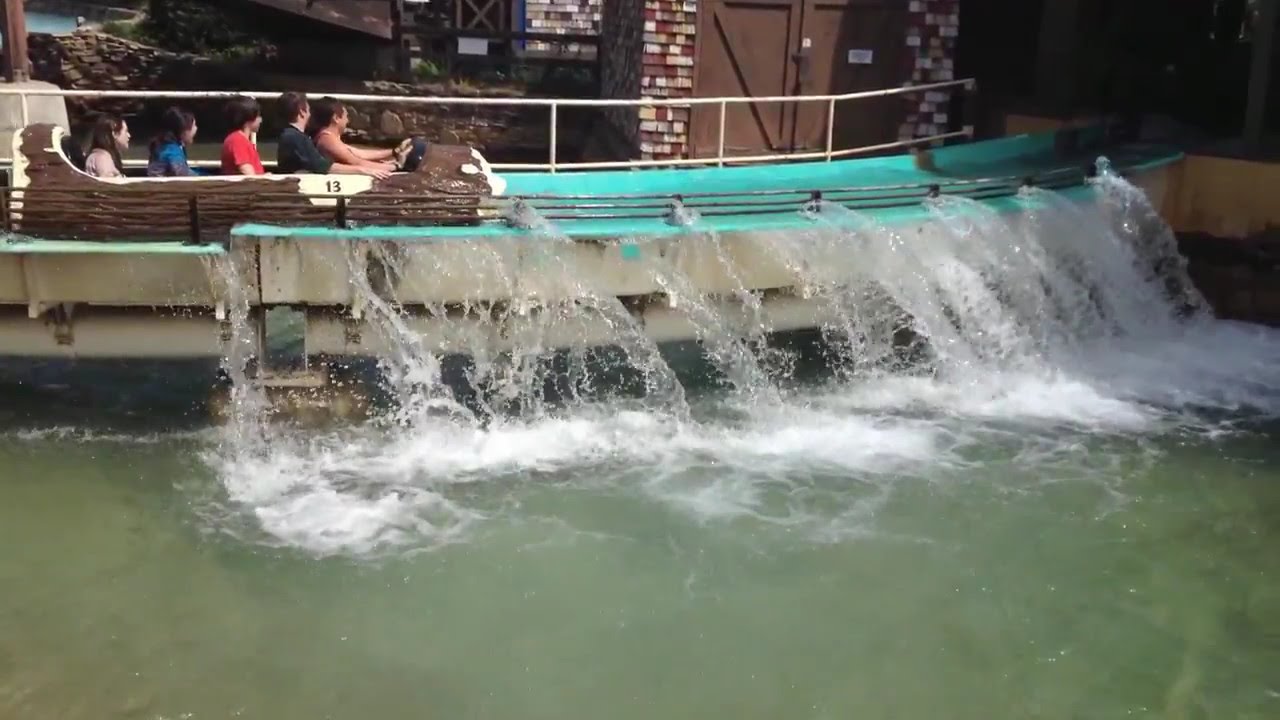The image depicts a vibrant scene at an amusement park, specifically capturing a water ride on a sunny day. Central to the photograph is a brown, log-shaped boat, crafted from plastic, carrying five cheerful riders along a curving water channel. Among the passengers are three women and two men, dressed in varying outfits: the person in the front wears a sleeveless purple top, the second wears a black t-shirt, the third dons a red t-shirt, the fourth is in a blue garment, and the fifth person at the back is in a pink sweatshirt. The log is marked with the number 13, and as it traverses the channel, water can be seen jetting out from the sides, cascading into a larger waterway on the right. The foreground features a visible rail alongside the channel, which guides the ride. In the backdrop, a faux rock wall and a couple of brown buildings are present, with one structure partially obscuring a darker area beyond. The light reflects the joy and exhilaration of the riders as the scene is brightened by clear, sunny weather.